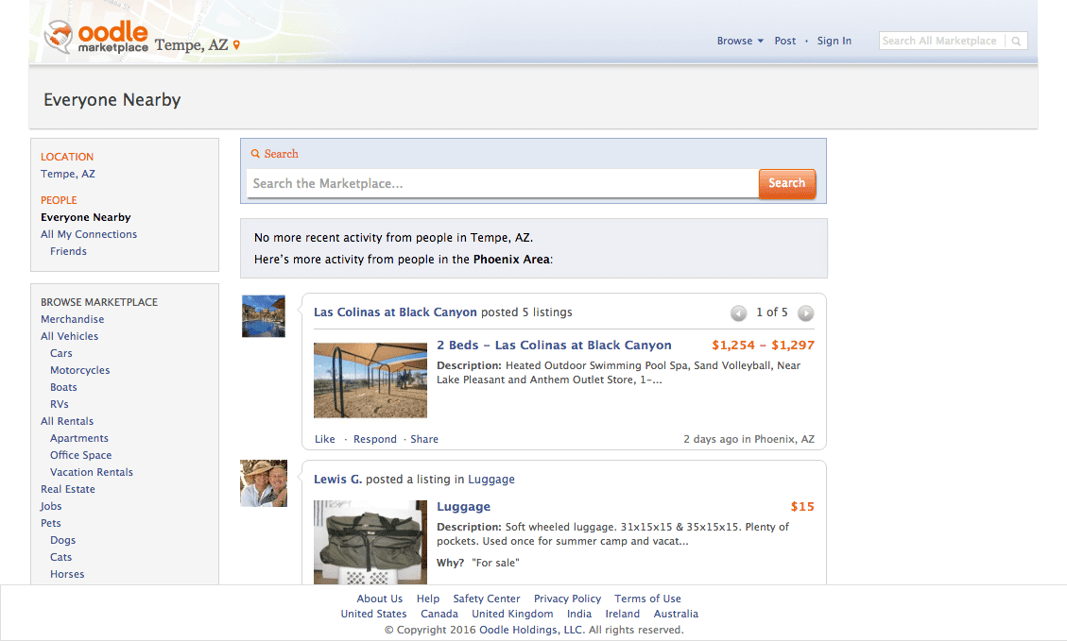In the top left corner of the image, the text "OODLE" is displayed in vibrant orange, followed by "Marketplace" just below it. The location "Tempe, Arizona" is prominently shown, with "Explore Nearby" in bold black text below it. Under the location, there are additional options such as "People, everyone nearby, all my connections, friends." To the right of these options, there's a search bar labeled "Search the Marketplace."

Below this is a message stating, "No More Recent Activity from People in Tempe, Arizona," followed by, "Here's more activity from people in the Phoenix area." 

Central to the image is a square picture of a playground, featuring a significant amount of sand and a swimming pool located in the upper left corner. 

Adjacent to this, details for a property named "Las Colinas at Black Canyon" are provided. The property, which includes two beds, is listed with a price range of $1,254-$1,297. Amenities mentioned include a heated outdoor swimming pool and a sand volleyball court, situated near Lake Pleasant.

Further down, a listing by Louis G. is highlighted in the luggage category, featuring an image of soft-wheeled luggage. The luggage is described as having plenty of pockets and being used only once for summer camp and vacation, with an explanation provided for its sale.